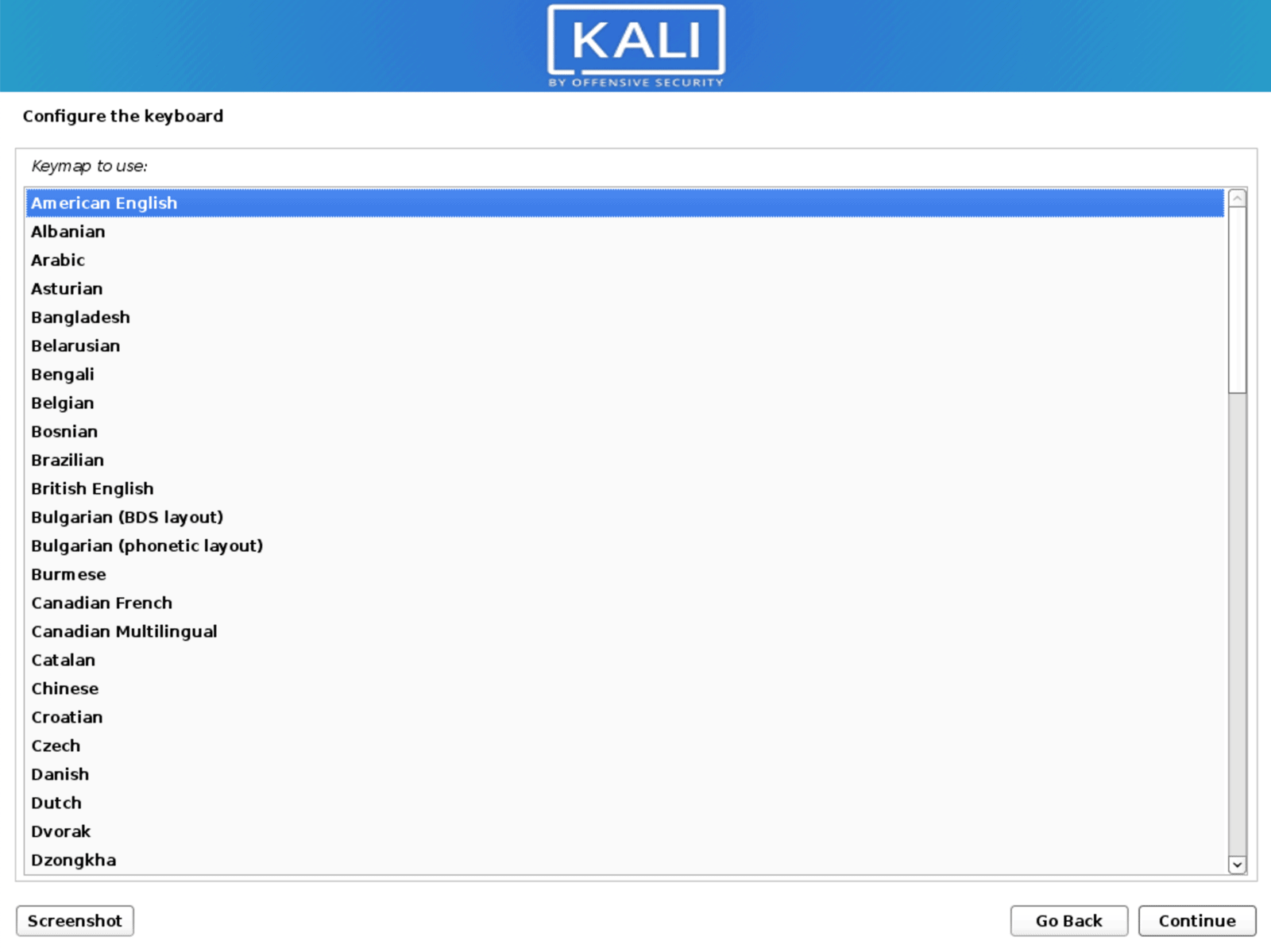The image displays a webpage with a prominent blue banner at the top. The banner's color gradient transitions from a lighter blue at the edges to a darker, blue-purple hue in the center. Centrally positioned on the banner is a square surrounding the bold, capitalized letters "KALI". Below this, the text reads "By Offensive Security". 

Beneath the banner, the phrase "Configure the Keyboard" is prominently displayed. Immediately below this, there is a square containing an extensive list of languages, with "American English" highlighted in the same blue as the banner, indicating an active selection. The list includes languages such as Albanian, Arabic, Asturian, Bangladeshi, Belarusian, Bengali, Belgian, Bosnian, Brazilian, British English, Bulgarian (both BDS and phonetic layouts), Burmese, Canadian French, Canadian Multilingual, Catalan, Chinese, Croatian, Czech, Danish, Dutch, Dvorak, and Dzungar.

At the bottom of the image, the options "Screenshot" in black text, "Go Back," and "Continue," both in black text within bordered boxes, are visible, indicating available navigation choices on the page.